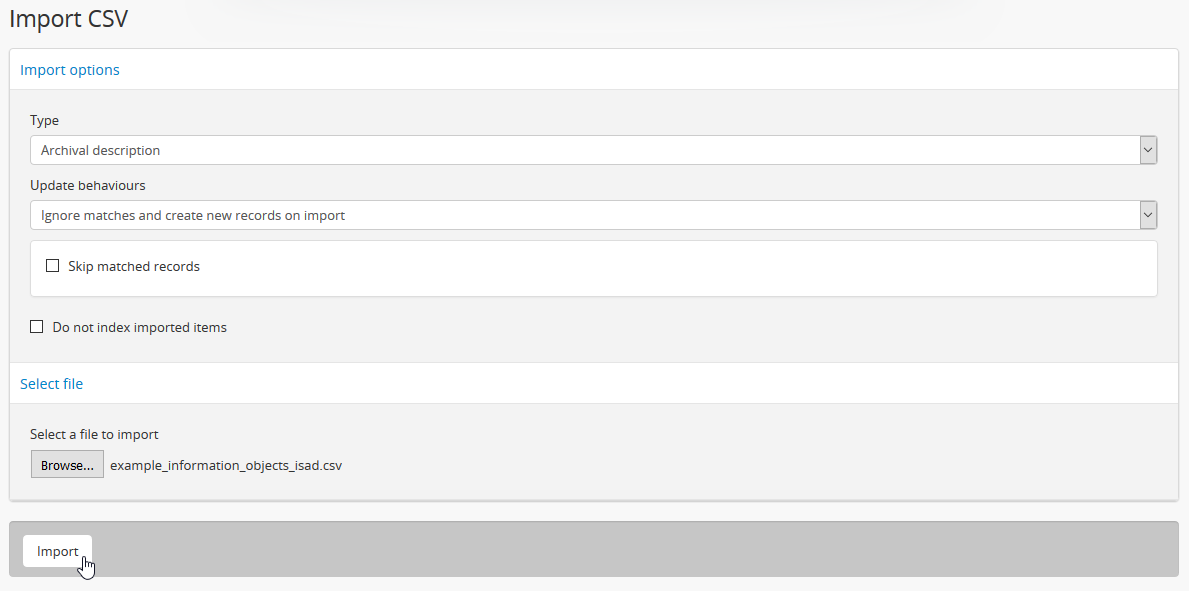The image features a light purple background. At the top, there is text that reads "Import CSV." Below this, there's a large white box with the heading "Import Options" in blue. Inside the white box, there is a section labeled "Type" with a dropdown menu that currently displays "Archival Description." Following this are update behavior settings reading, "Ignore matches and create new records on import," also accompanied by a dropdown arrow.

Next is another white box that contains small checkboxes with the options "Skip matched records" and "Do not index imported items" in blue text. A subsequent white box has the label "Select file in Blueprint," followed by a blue box containing the instruction "Select a file to import" and a "Browse" button. The example names listed include "Information," "Objects," and another obscured item.

At the bottom of the setup, there's a prominent "Import" button resting on a purple background.